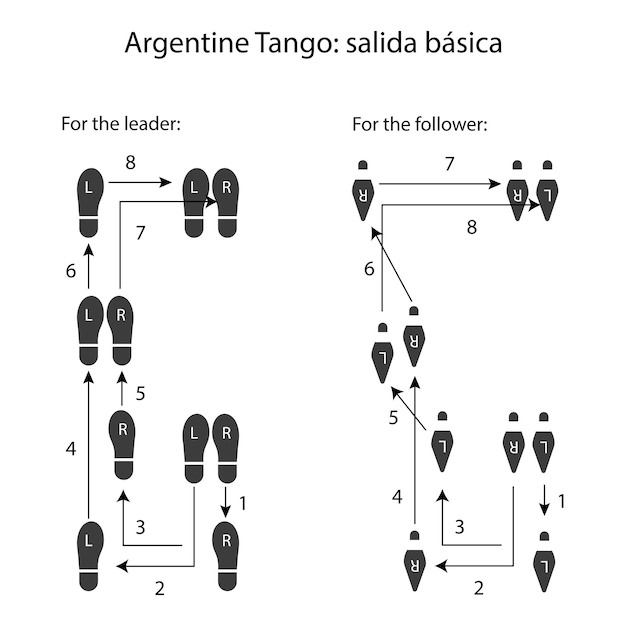The image is a detailed step-by-step guide for dancing the Argentine Tango, specifically the "Salida Básica." At the top, it reads "Argentine Tango: Salida Básica." The diagram is divided into two halves: the left side for the leader and the right side for the follower. The leader's steps are shown with footprints resembling male shoes, starting from the bottom with the feet together. The sequence involves the right foot stepping back on one, the left foot stepping to the left, and the right foot moving forward, amongst other steps, up to eight. Meanwhile, the follower's steps, which mirror the leader's pattern, are depicted upside down with footprints resembling female heels, indicating the follower is facing the leader. The follower's movements also include eight steps, showing where each foot should be placed and how they align with the leader's steps. Despite the overall symmetry, steps five and six differ between the leader and the follower, highlighting a key variation in their movements. Arrows and numbered steps guide the dancers through the routine, making the instructions clear and detailed.